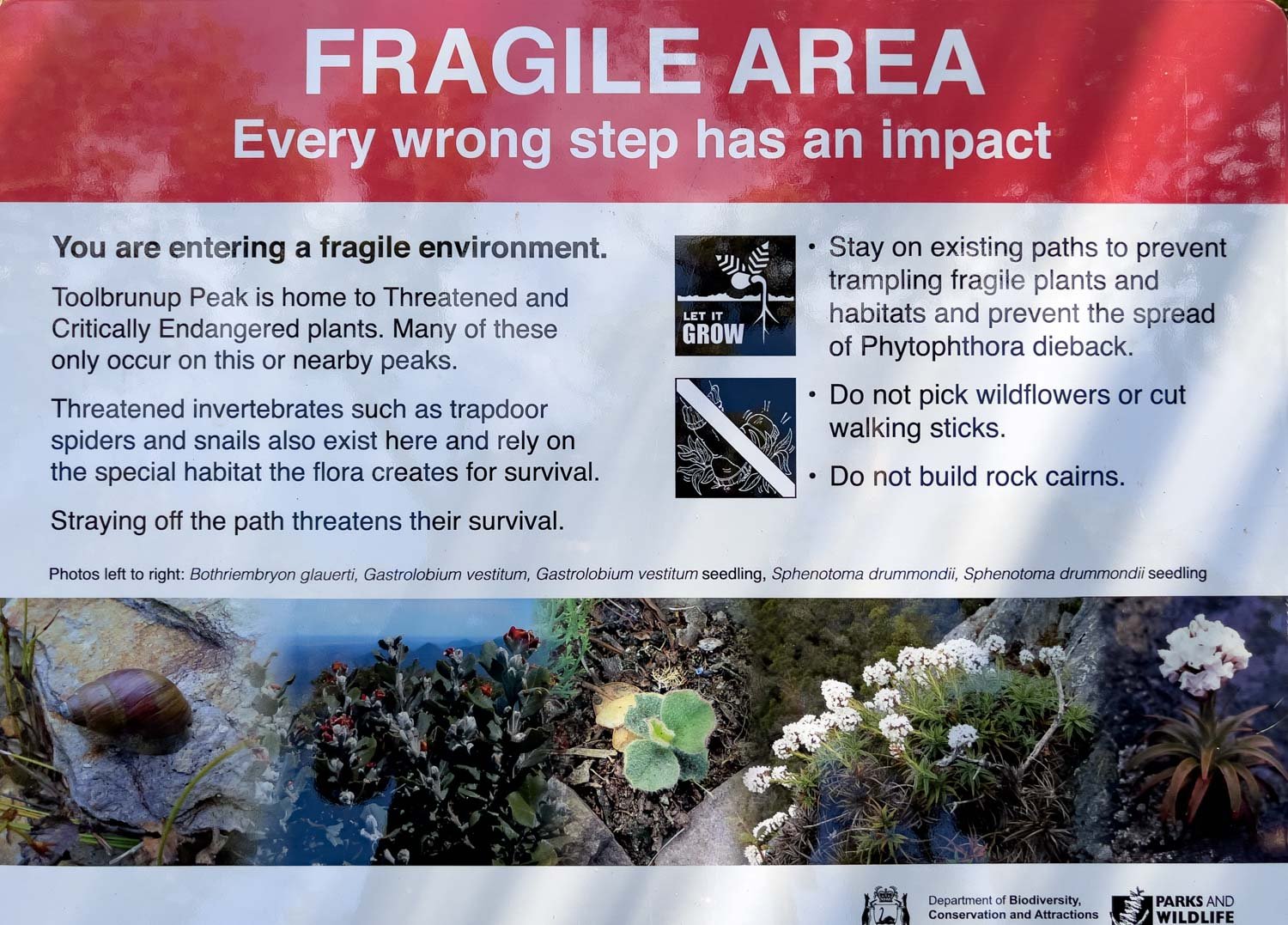The sign prominently displays a warning at the top, with white text on a red background stating, "Fragile Area. Every wrong step has an impact." The central section features black text on a white background, explaining, "You are entering a fragile environment. Two Brunette Peak is home to threatened and critically endangered plants, many of which are unique to this and neighboring peaks. Threatened invertebrates like trapdoor spiders and snails also inhabit this area, relying on the special habitat the flora provides for survival. Straying off the path threatens their survival." The right side of the sign instructs, "Stay on existing paths to prevent trampling fragile plants and habitats and to prevent the spread of Phytophthora dieback. Do not pick wildflowers or cut walking sticks. Do not build rock cairns." At the bottom, there are pictures showcasing the endangered plants and invertebrates mentioned. The sign underscores the importance of adhering to these guidelines to protect the delicate ecosystem.